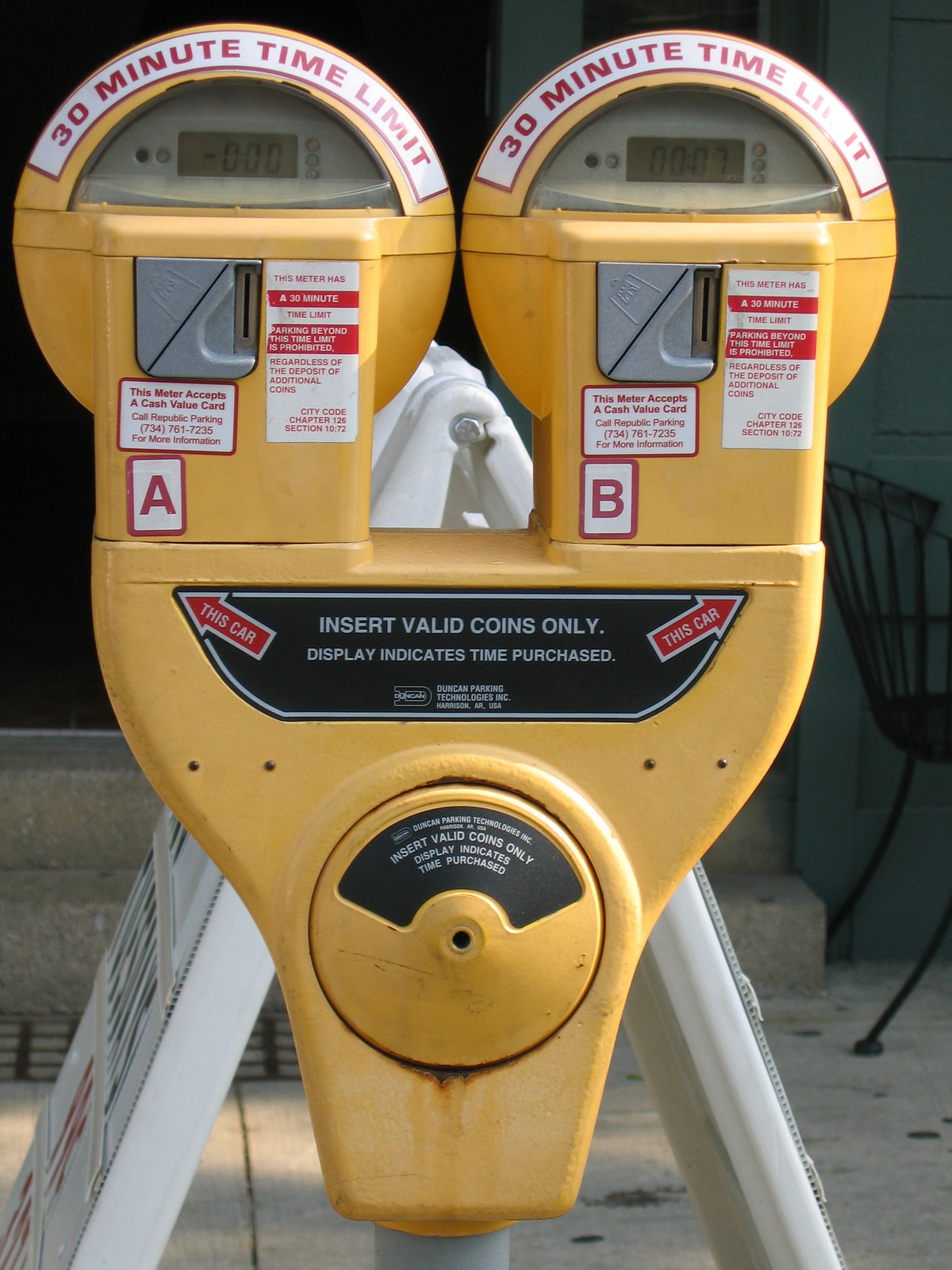This detailed image features a bright yellow parking meter during the day, capturing a close-up view. The meter is approximately 50% taller than it is wide and designed for two vehicles, marked with a letter "A" on the left meter and "B" on the right. Both meters are equipped with digital displays, showing times of 0 and 7 minutes respectively. The top curved portion of each meter prominently displays a white band with red text reading "30 minute time limit." Below this, each meter has instructions and labels in black, white, and red. Notably, a large black label stretches across the bottom part of the meter, instructing "insert valid coins only" alongside red arrows pointing left and right, with additional text specifying that the display indicates the time purchased.

In the background, to the right, a black chair with black legs sits against a dark teal-green wall. Behind the meter, there is a structure featuring grey steps and a lined black grate at the base, leading towards a black door. Additionally, there is a white sandwich board sign in a V-shape with unclear red and black lettering positioned behind the parking meter. The sidewalk beneath shows signs of wear with visible splotches. The overall scene indicates a typical urban environment, with the intricate details of the parking meter standing out.